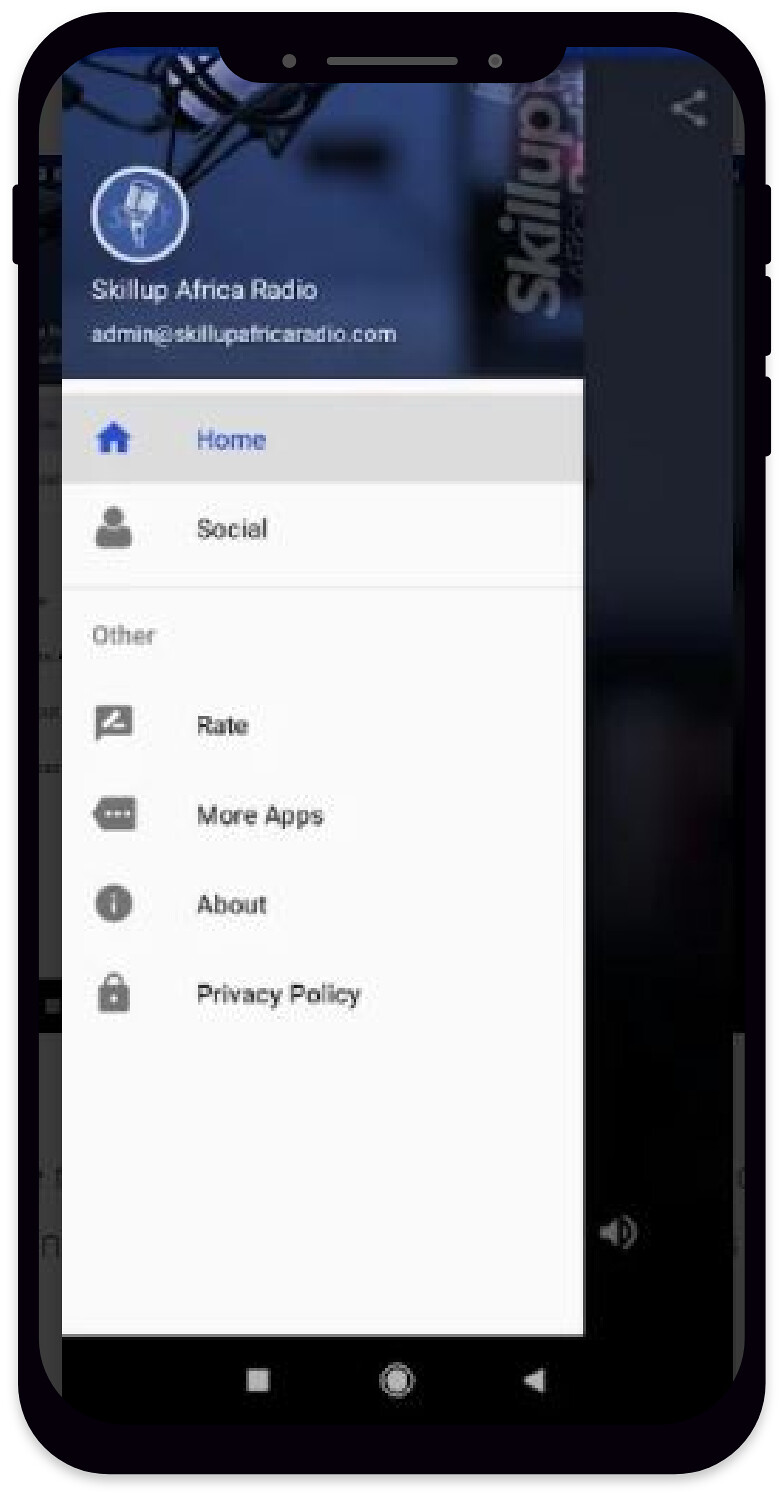**Caption:**

A black smartphone displays a detailed navigation menu on its screen. The device features three buttons along the upper right side and one button on the upper left. The top section of the screen has a vibrant blue header with the text "Skill Up" aligned to the right. Adjacent to this, on the left, is a blue logo above the white text "Skill Up Africa Radio," accompanied by the email address "admin@skillupradio.com" beneath it.

The primary menu area is white and prominently lists several options. At the top is "Home," marked by a small home icon to its left. Directly beneath "Home," which is highlighted with a gray outline and blue text, are additional menu items in gray text: "Social" paired with a person icon, "Rate" associated with a somewhat unclear symbol, "More Apps" denoted by an arrow and three dots, "About" indicated by a circle with an eye, and "Privacy Policy" marked with a lock icon.

The intricate menu layout and distinctive icons provide a comprehensive and user-friendly interface for navigating Skill Up Africa Radio's features.